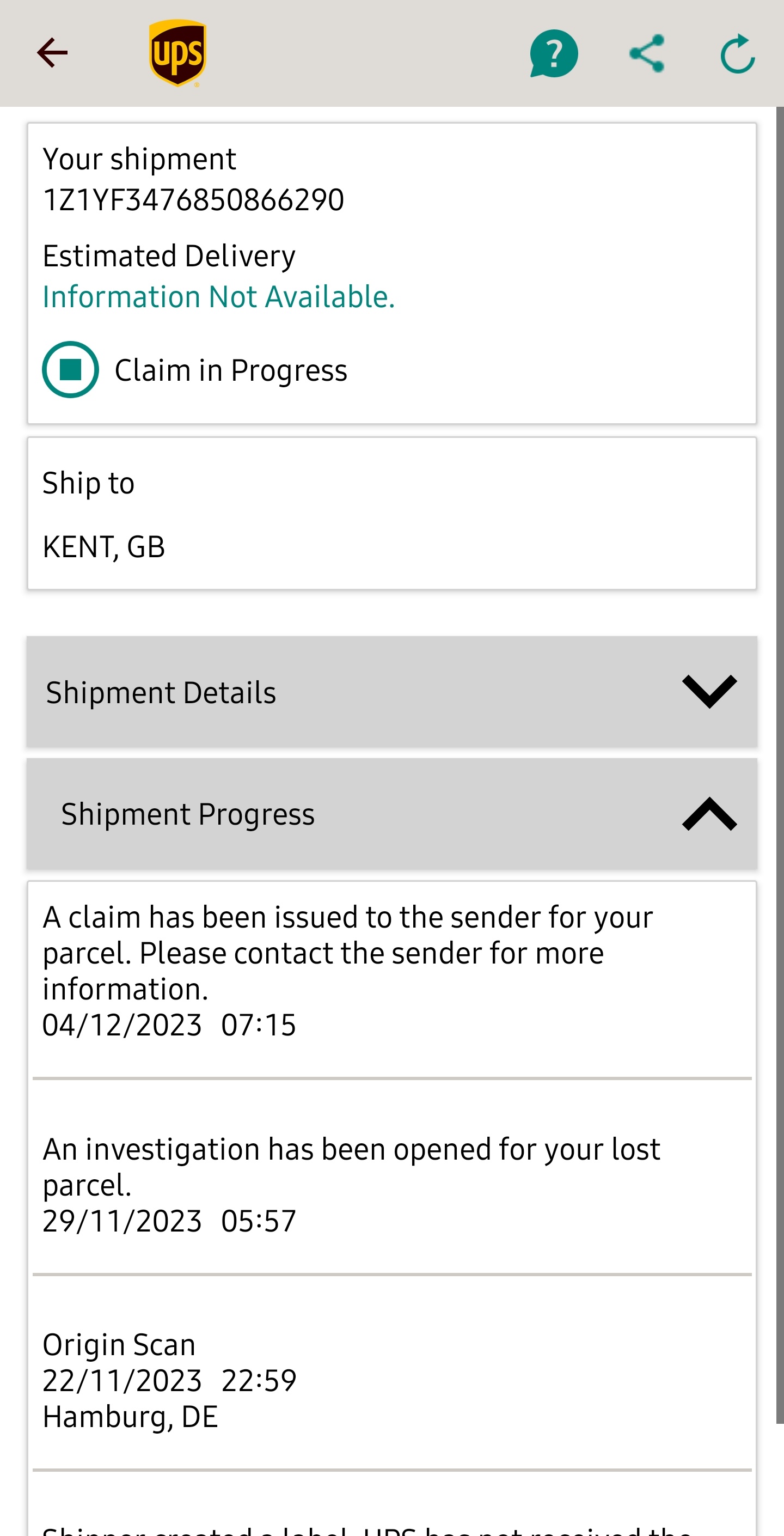This detailed caption describes the element present in a UPS shipment result screenshot image:

The screenshot displays the progress of a UPS shipment. At the top, there is a gray-colored navigation bar featuring an arrow to go back, the UPS logo, and options for sharing and accessing additional information. Below, a box presents the shipment number and the estimated delivery details.

Another section indicates the delivery destination as Kent, GB. Directly beneath, there is a section for shipment details, which is currently collapsed. The open shipment progress section reveals that a claim has been issued to the sender, instructing the recipient to contact the sender for more information. This notice is dated April 12, 2023, at 7:15 AM.

Further down, an entry dated November 29, 2023, at 5:57 AM mentions that an investigation has been opened for the parcel. The origin of the shipment is documented with an origin scan from Hamburg, DE, recorded on November 22, 2023, at 10:59 PM.